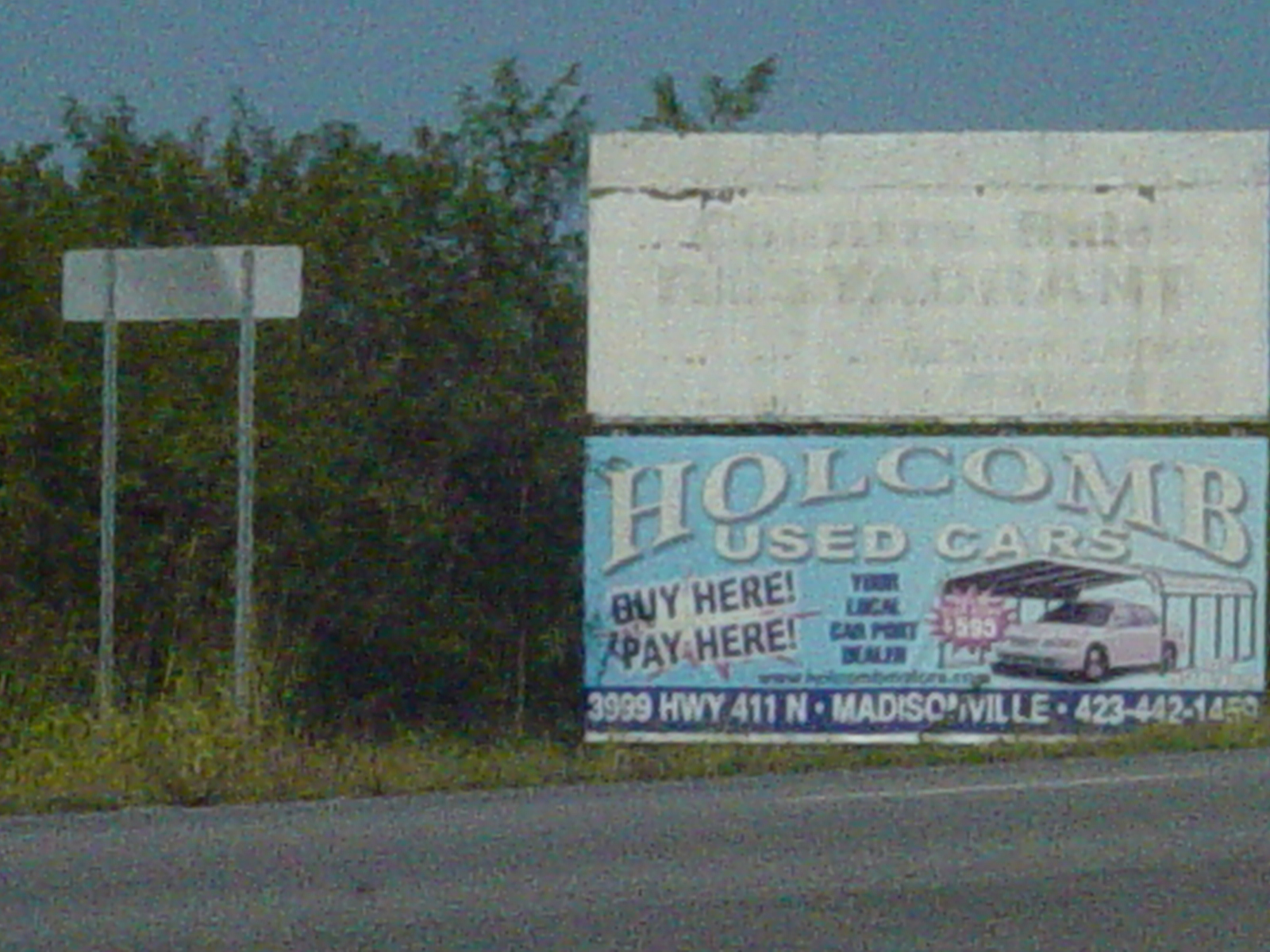A grainy photograph captures a desolate stretch of road flanked by two prominent billboards and an indiscernible street sign. In the foreground lies a paved road leading the eye to the primary focus of the image: two billboards. The upper billboard is blank, bearing only faint hints of previously displayed content that has either faded over time or been removed entirely. Below, at ground level, a more vibrant billboard with a light blue background advertises "Holcombe Used Cars." The text reads "buy here, pay here," accompanied by an image of a sedan parked below a small canopy roof. Although the photograph's quality obscures finer details, there's an indication of additional text that is largely unreadable, possibly displaying a price related to either the car or the canopy. The address "3999 Highway 411 North, Madisonville" and a partially legible contact number "423-442-14" are also visible. Surrounding the billboards is a mix of greenery, including trees and grass, with an unreadable road sign facing away from the camera, adding to the overall rustic and slightly neglected atmosphere of the scene.